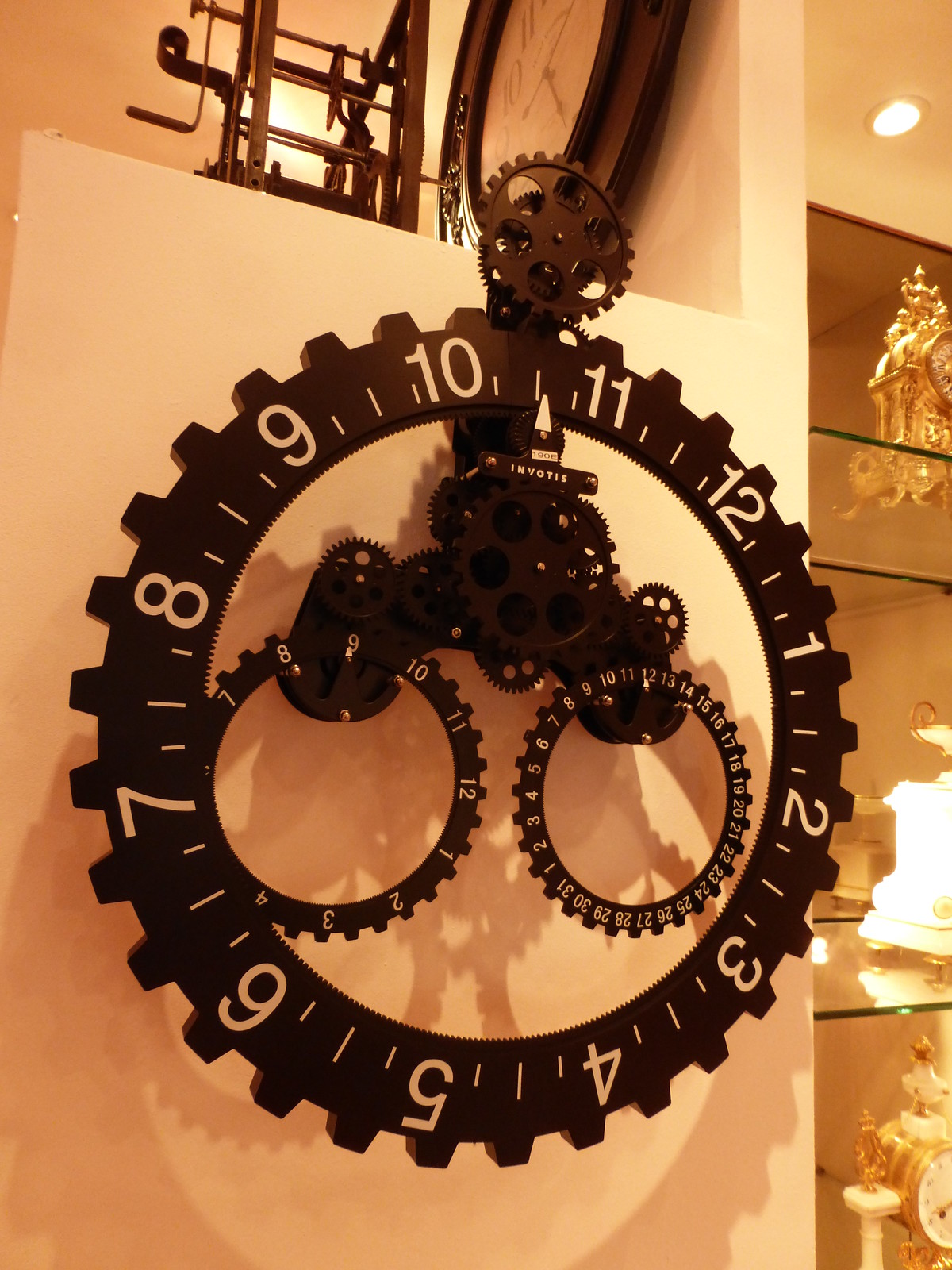This color photograph showcases an intriguing and non-traditional clock design mounted on a white wall, crafted with interconnected gears and cogwheels. The outer perimeter features a large toothed ring gear with numbers 1 through 12 in a clockwise sequence, though somewhat unevenly spaced, with 10 and 11 positioned near the top. A triangular pointer is located inside the top of this outer gear. Inside the larger gear, there are two smaller, numbered cogwheels: one marked 1 through 12 on the left, and another marked 1 through 31 on the right, possibly indicating a calendar function. These components are all part of a mechanical system that includes a gear at the top with cut-outs, allowing it to rotate. The clock's hour hand is an upward-pointing arrow on a gear mechanism. The brand name "INVOTIS" is prominently displayed on a larger gear within the assembly. To the right of this clock, a glass display cabinet holds various decorative items, including what appear to be antique clocks on its top and bottom shelves.